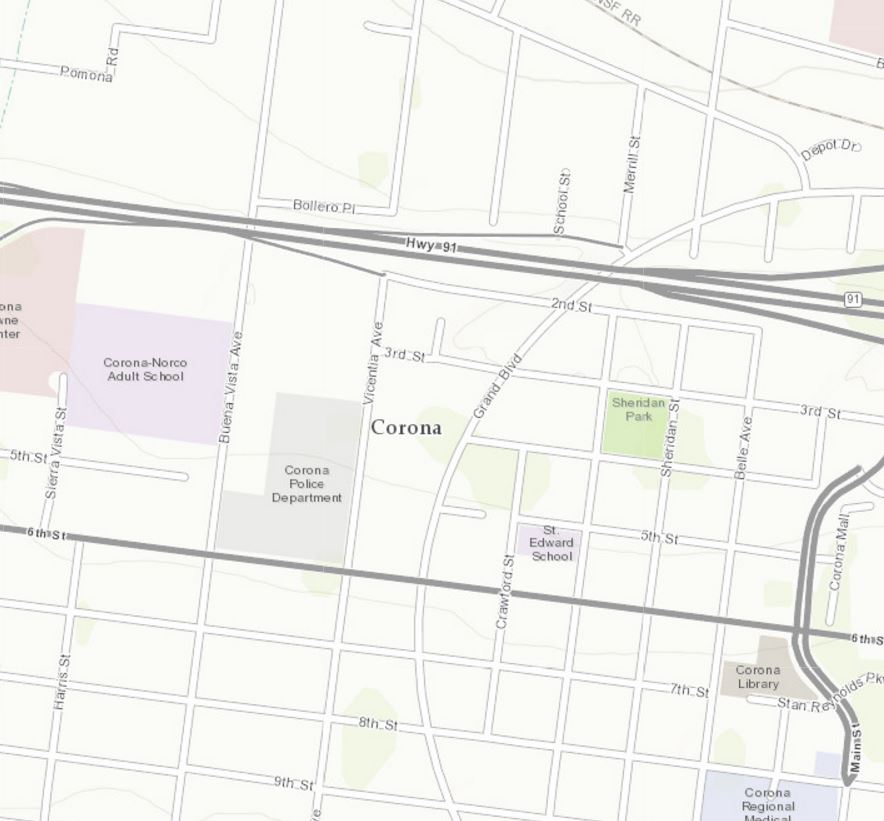This detailed map of Corona meticulously highlights prominent locations with distinctive color coding for easy identification. Featured landmarks include the Corona Norco Adult School, Sheridan Park, Corona Library, Corona Mall, Corona Regional Medical Center, and St. Edward School. The map also shows the Stan Reynolds Parkway and clearly depicts Highway 91 skirting the edge of the town. Every street within the town is labeled, ensuring no road goes unidentified. Main Street, along with the mall situated right on it, is prominently marked. The map offers a comprehensive and navigable layout of Corona’s intricate network of streets and significant places of interest.